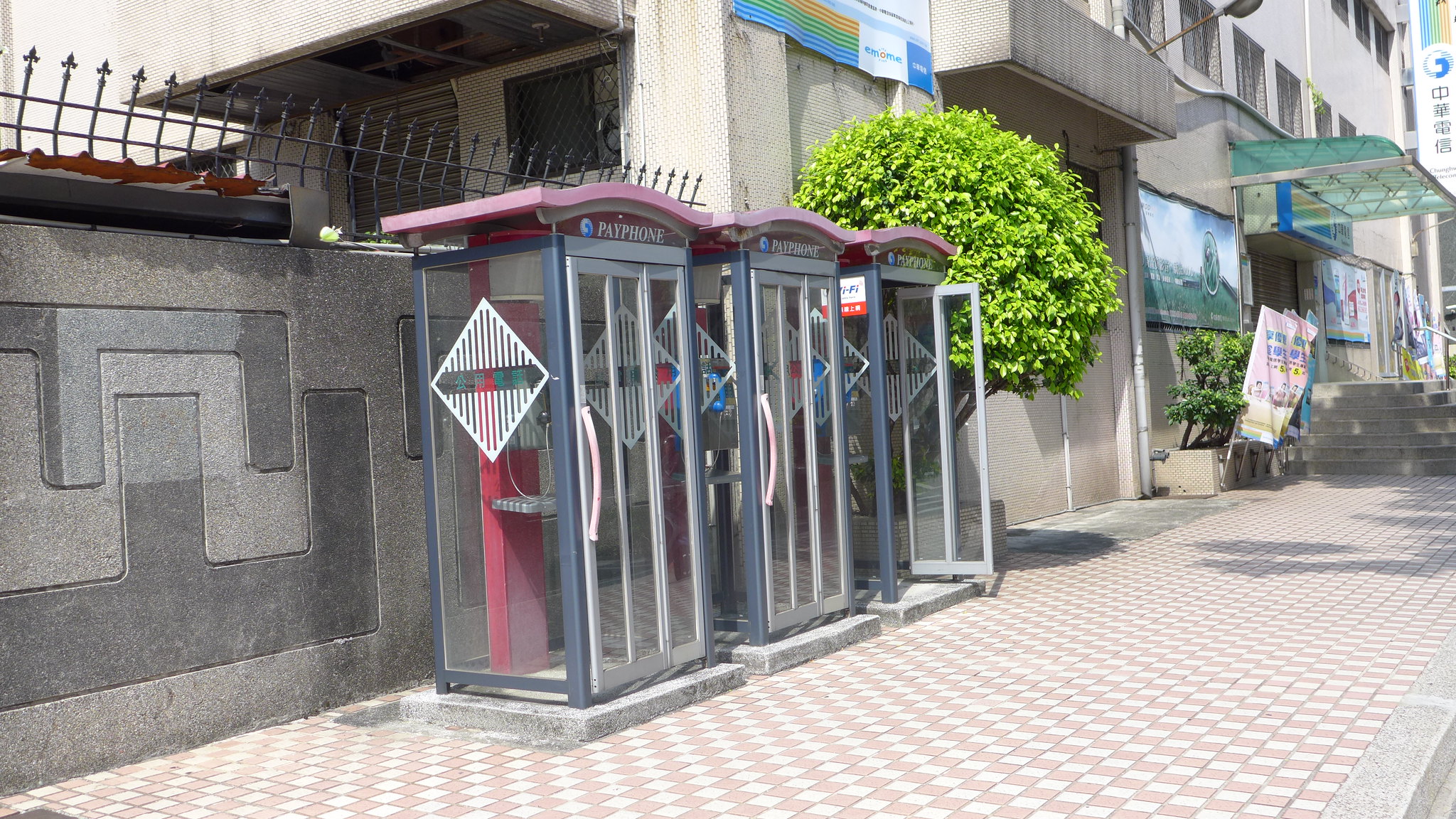The photograph captures a dynamic city street scene from the perspective of someone standing at the edge of a pink-and-white checkered brick sidewalk. The sidewalk's small, alternating squares create a diamond pattern as it stretches down the length of the street. Adjacent to this sidewalk is a granite wall adorned with geometric, boxy grooves, enhancing the modern cityscape. Along this wall, there are three identical phone booths, each completely encased in clear glass, standing in a row. These phone booths feature red roofs and doors with long curved handles that bend slightly when opened. The doors and walls are transparent, allowing a full view inside, where a red panel houses the phone.

Adding to the scene's architectural interest, the top of the granite wall is crowned with a spiked wrought-iron fence, suggesting the presence of an elevated walkway on the second floor of the building. A verdant, blossoming tree stands just to the left of the phone booths, providing a touch of nature amidst the urban environment. Further down the street, the storefronts continue, including one with a green awning jutting out, hinting at a bustling commercial area.